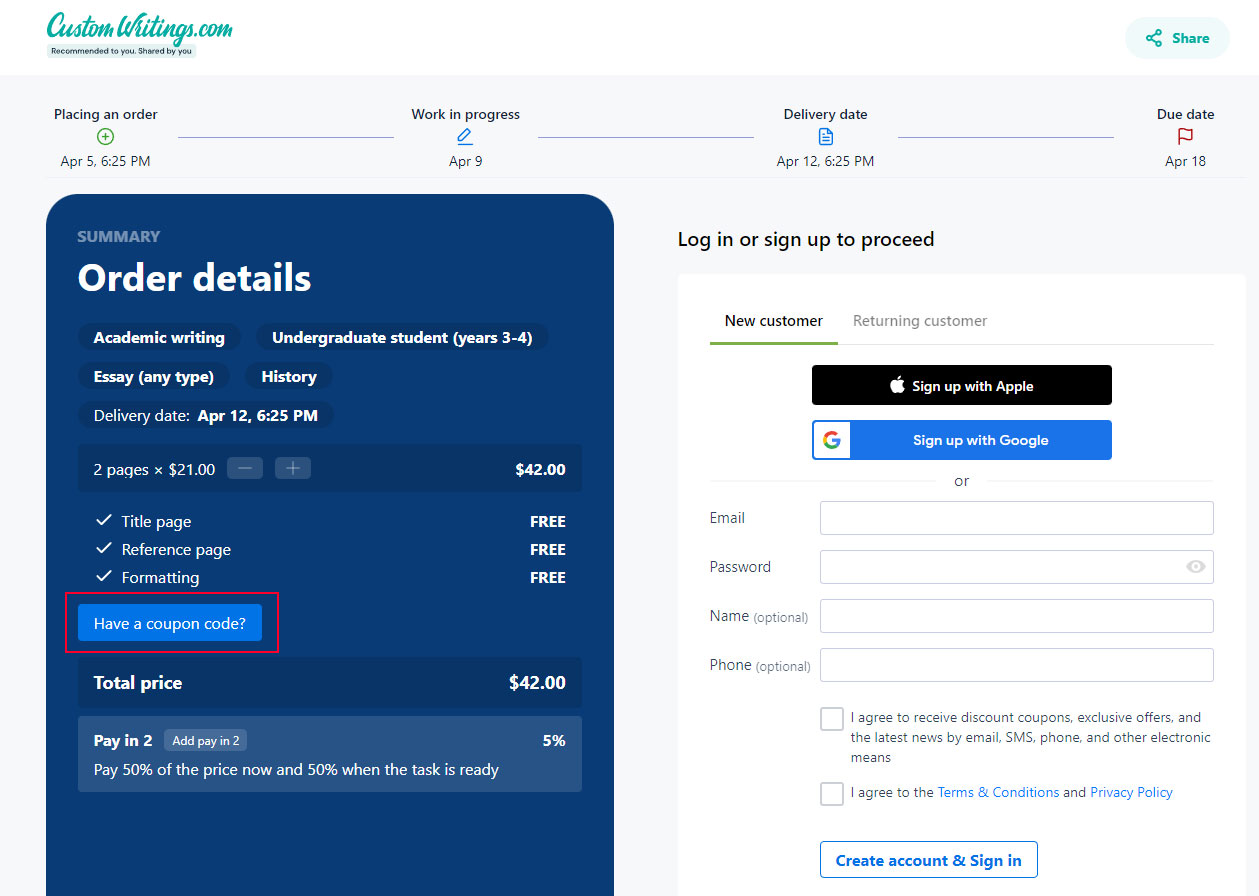The image depicts a screenshot from the website CustomWritings.com, identifiable by its dark indigo-colored logo situated in the top left corner. The screen showcased here is the checkout page, where the main focus is on a dark blue square window on the left side titled "Summary Order Details." This window details the order, stating that two pages cost $42, which also reflects the total price. Below this, there is a prominent red-outlined rectangle surrounding a blue button labeled "Have a Coupon Code." 

To the right of this window, the interface offers sign-in options via Apple and Google, each represented by distinct buttons. The website's background is predominately white, providing a clean and simple layout. At the top of the page, a horizontal timeline indicates the order progress, highlighting phases from order placement to work in progress, along with the delivery and due dates.